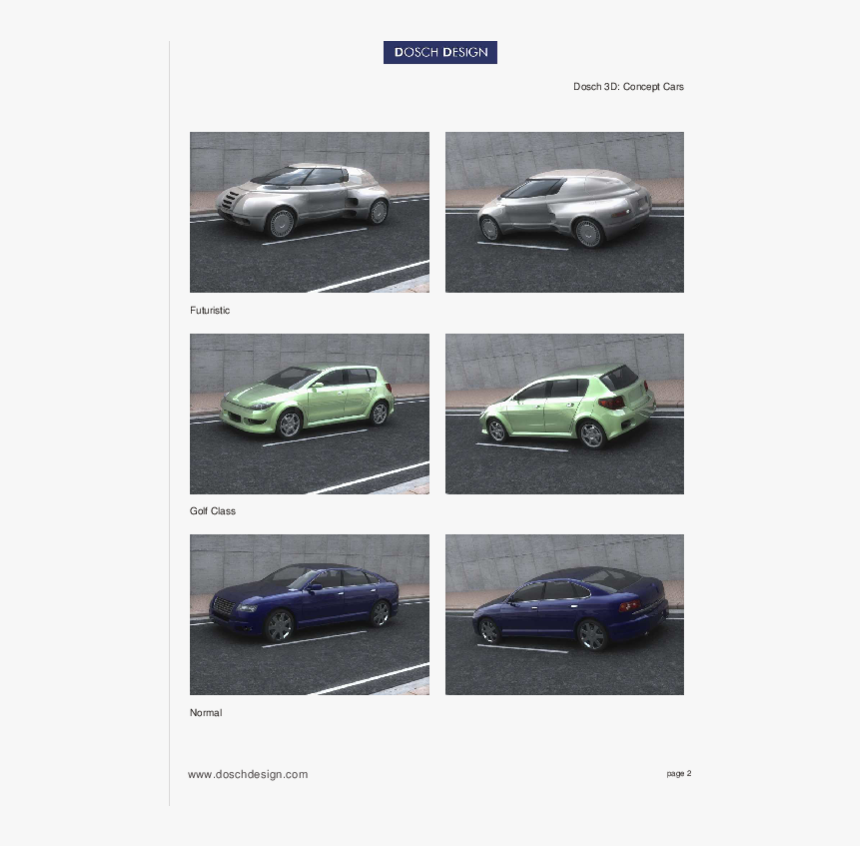A sleek gray background serves as the canvas for the design concept on display. Central to the composition is a Blu-ray rectangle featuring the white, 3D "DASH" logo prominently. The visual presentation is divided into three rows, each showcasing different concept cars.

- The first row features two futuristic cars rendered in grayscale, embodying advanced design and innovation.
- The second row presents two green vehicles labeled "golf class," reflecting eco-friendly and sporty attributes.
- The third row features two blue cars labeled "normal," highlighting practical and everyday usability.

At the bottom of the image, the website address "www.dashdesign.com" is clearly displayed, providing a point of reference for further information. Additionally, towards the right side of the image, the text "Page 2" indicates that this is part of a larger series or presentation.